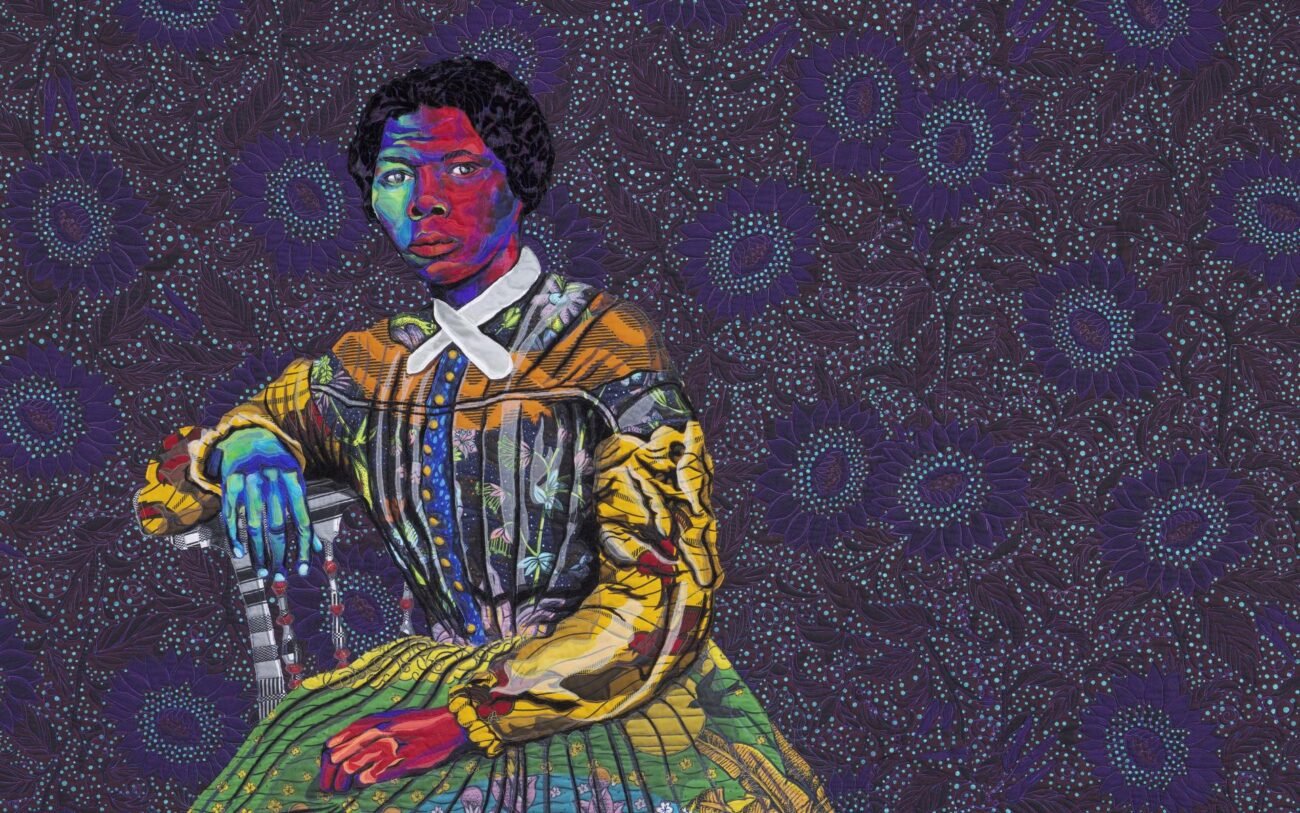The image is a vibrant, abstract color painting by artist Bisa Butler, featuring African-American historical figure Harriet Tubman. The painting, in landscape orientation, shows Tubman seated on the left side, facing the viewer with a neutral expression. Her skin appears illuminated with a blend of multiple colors: the right side of her face is bathed in bluish hues transitioning to red, while the left side has a magenta and orange palette, accented by turquoise and green. Tubman's large, wide nose and lips are distinctive features of her African-American heritage. Her hands also showcase this colorful variation; her left hand (resting on her lap) glows with magenta and orange hues, while her right hand, draped over the back of a chair, is blue.

She is wearing a long-sleeved, multicolored dress with vertical stripes, featuring gold puffy sleeves and a white crisscross scarf at the neck, and a skirt gathered at the waist. Her black hair is pulled back neatly. The background of the painting is a dark burgundy shade, embellished with abstract blue flower shapes and scattered white dots, contributing to the overall dynamic and emotive composition of the artwork.